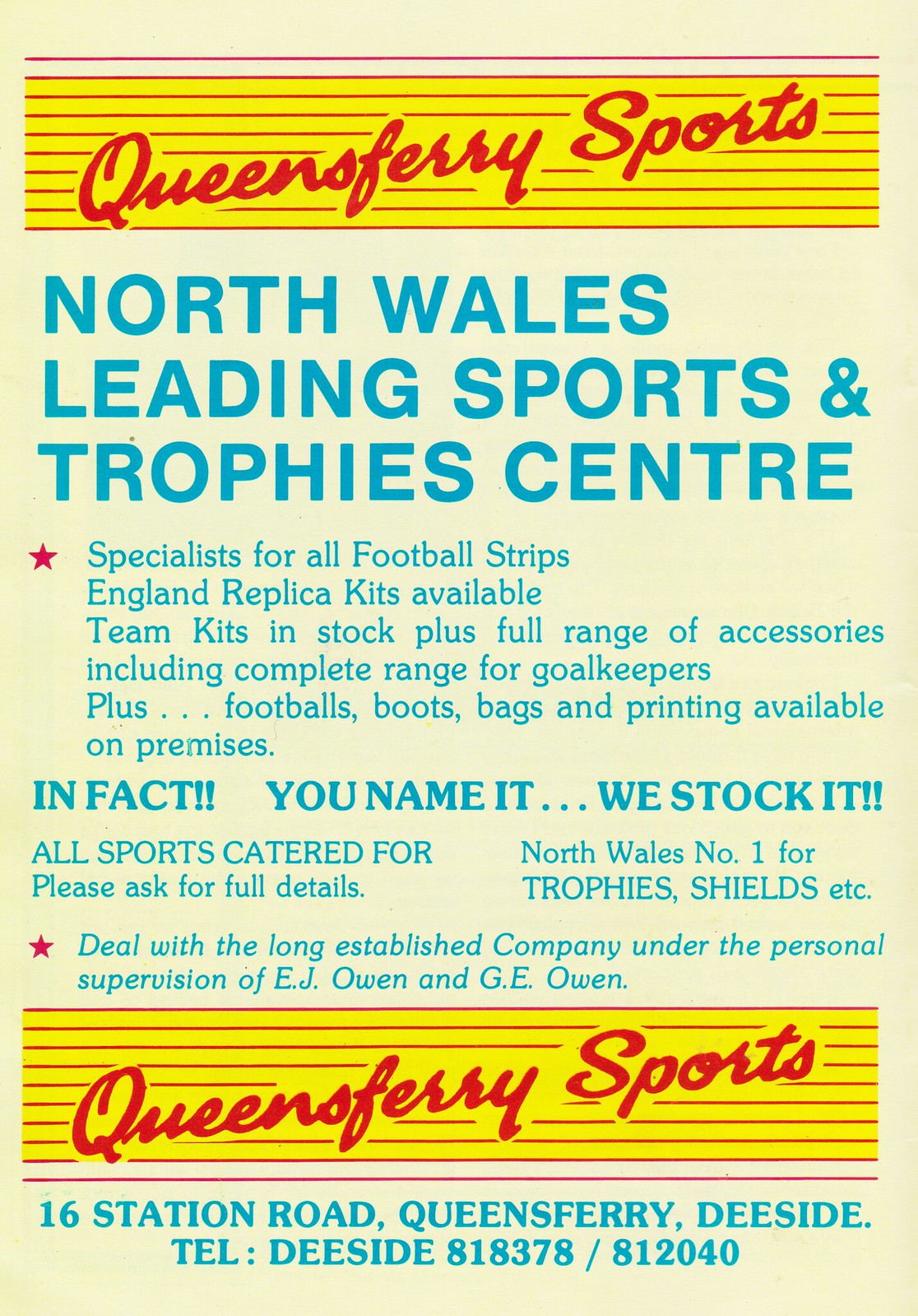The image is a rectangular advertisement for Queensferry Sports, featuring a background of cream or light yellow adorned with red horizontal stripes at the top and bottom. The shop's name, "Queensferry Sports," is prominently displayed in red, scrolled text on a yellow band. Below this, in blue capital letters, it reads, "North Wales Leading Sports and Trophy Center." The advertisement highlights the store’s offerings: specialists in all football strips, England replica kits, team kits in stock, and a full range of accessories including items for goalkeepers, footballs, boots, bags, and on-premise printing services. The ad claims, "In fact, you name it, we stock it," and emphasizes that "all sports are catered for," encouraging customers to ask for full details. It also boasts being "North Wales' number one for trophies, shields, etc." The business is described as long-established, operating under the personal supervision of E.J. Owen and G.E. Owen. The contact details, printed at the bottom in blue, list the address as 16 Station Road, Queensferry, Deeside, and the telephone number as Deeside 818-378-812040.